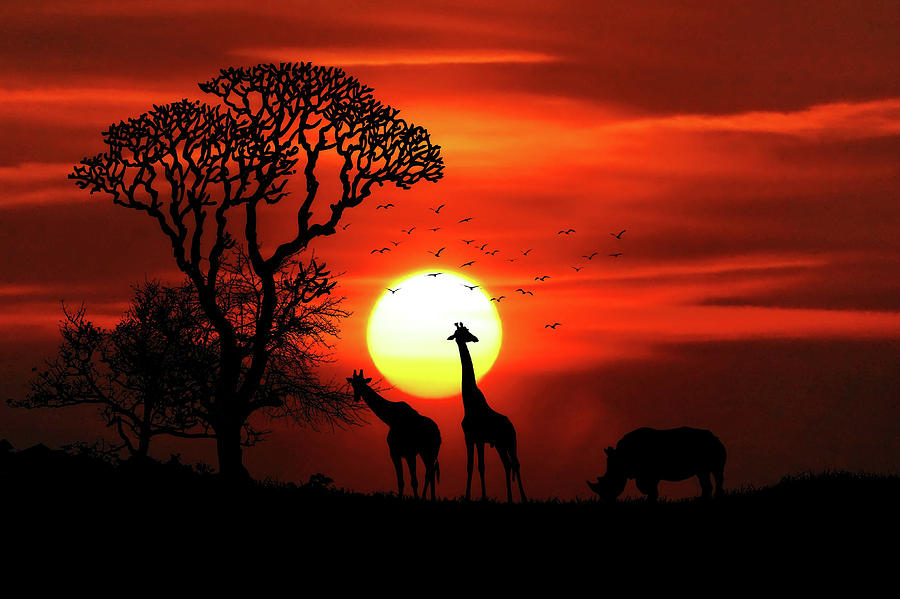This image is a stunning depiction of an African Savannah at either sunrise or sunset. Dominated by a deep, rich crimson sky, the image features various shades of red that transition into a brilliant, almost blinding white and yellow sun positioned slightly below the center. Silhouetted against this vivid backdrop, the foreground is entirely black, emphasizing the striking outlines of the landscape and wildlife.

Towards the bottom of the image, three animals stand out: two giraffes and one rhinoceros. One giraffe, its long neck and head crossing into the sun's glow, reaches up to nibble on the sparse leaves of one of two trees on the left, while the other giraffe leans down to graze from the tree’s lower branches. Meanwhile, the rhinoceros, situated further right, appears to be grazing off the ground. Above them, a flock of birds, possibly around twenty, is scattered across the sky near the sun, adding a dynamic element to the scene.

The branches of the two trees, extending long and thin, frame the image gracefully, adding to the sense of depth and scale. Various wispy clouds lightly streak across the sky, serving more to enhance the vibrant backdrop rather than obscure it. This beautifully fabricated image captures the essence of an African sunset, with silhouetted wildlife and dramatic natural hues combining to create a timeless and evocative scene.